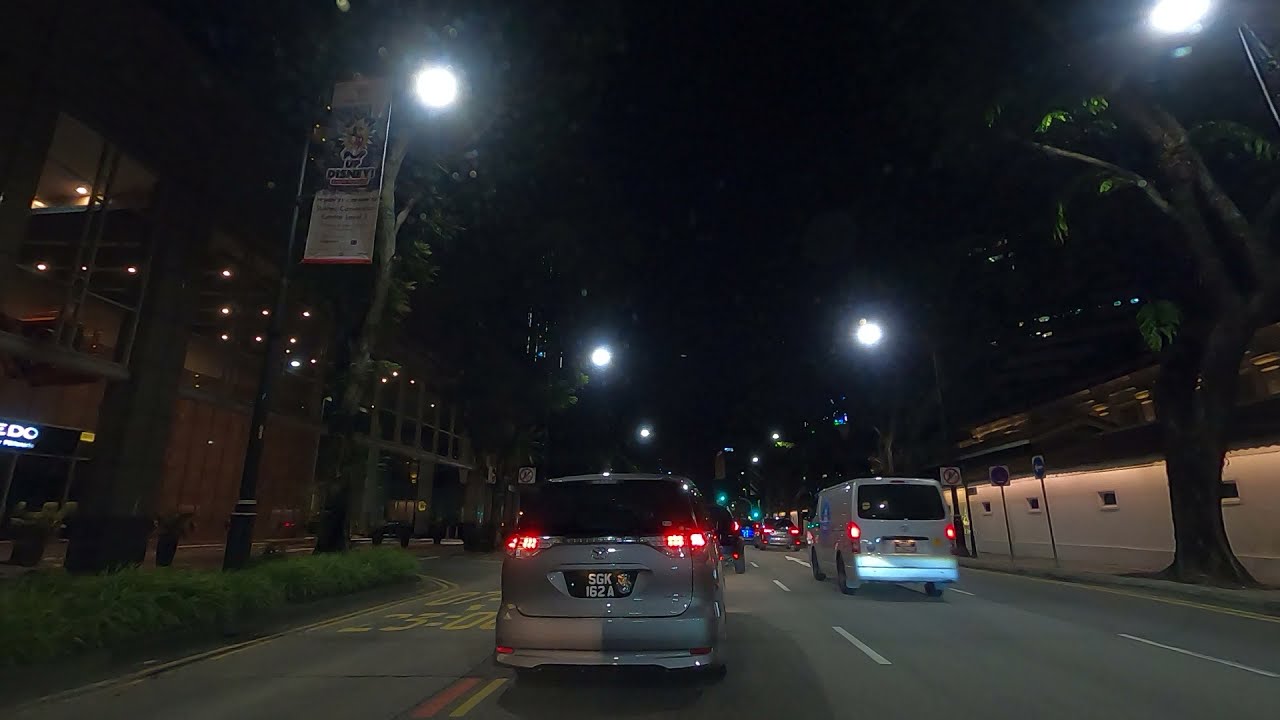This nighttime image captures a dark street in a European city, likely taken from a dash cam, given the perspective. The street features a line of vehicles traveling away from the camera, including a white cargo van on the right and a minivan on the left, with a discernible license plate reading SGK 162A. The four-lane road is partially empty, with the leftmost lane possibly designated for turning. Illuminated by streetlights, the scene reveals additional elements: a tree accompanied by multiple road signs, including a no-parking sign, on the right sidewalk, alongside some indistinguishable signs. The left side displays larger buildings with poles bearing somewhat legible, possibly foreign-language advertisements. The image is clear but devoid of any noticeable pedestrians, highlighting a serene but somewhat bustling urban environment.